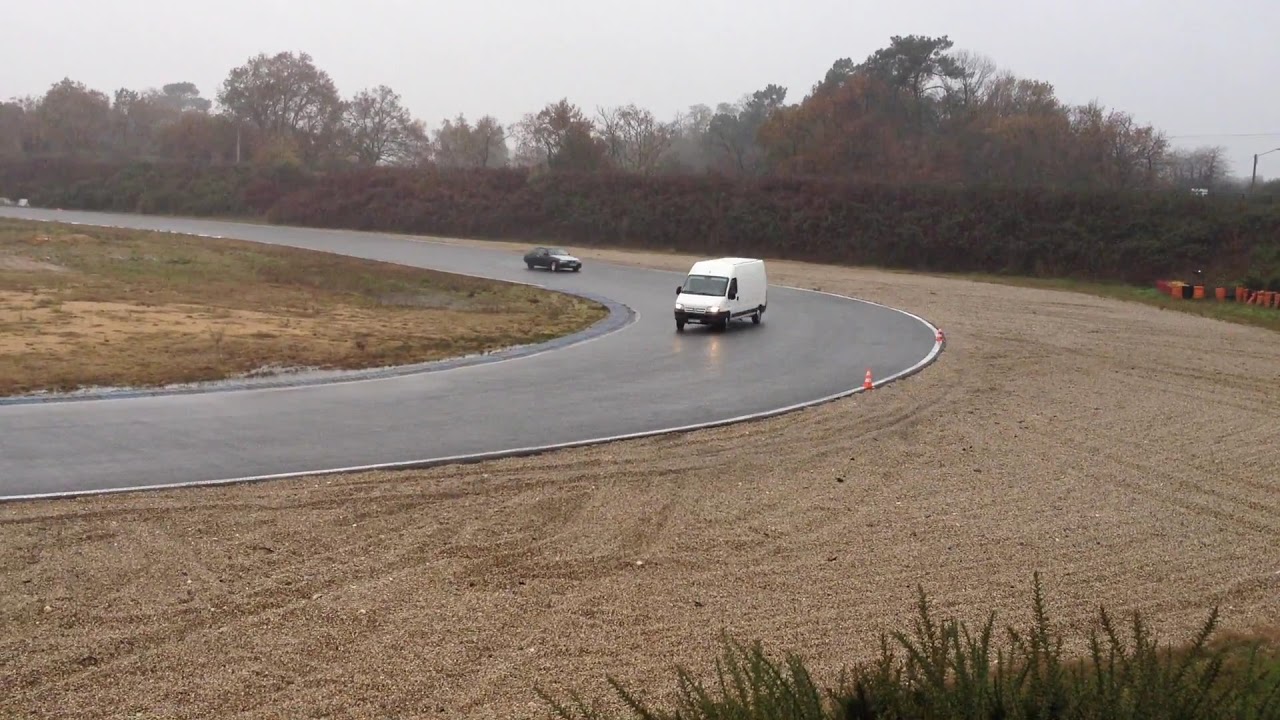A photograph captures a dreary, overcast day with a white utility van leading a curve on a dark gray asphalt road, followed closely by a black sedan. The wet, freshly completed road curves gently from the left to the center and then back to the left, headed towards the bottom right corner of the image. Orange and white traffic cones dot the curve, alongside some additional orange equipment near the tree line. To the left of the road, patches of grass and small bushes thrive, while the right side shows rich dark brown sand and gravel, marked by tire tracks. Tall bushes and trees with changing autumn leaves form a colorful backdrop, beneath a cloudy, rain-threatening sky.